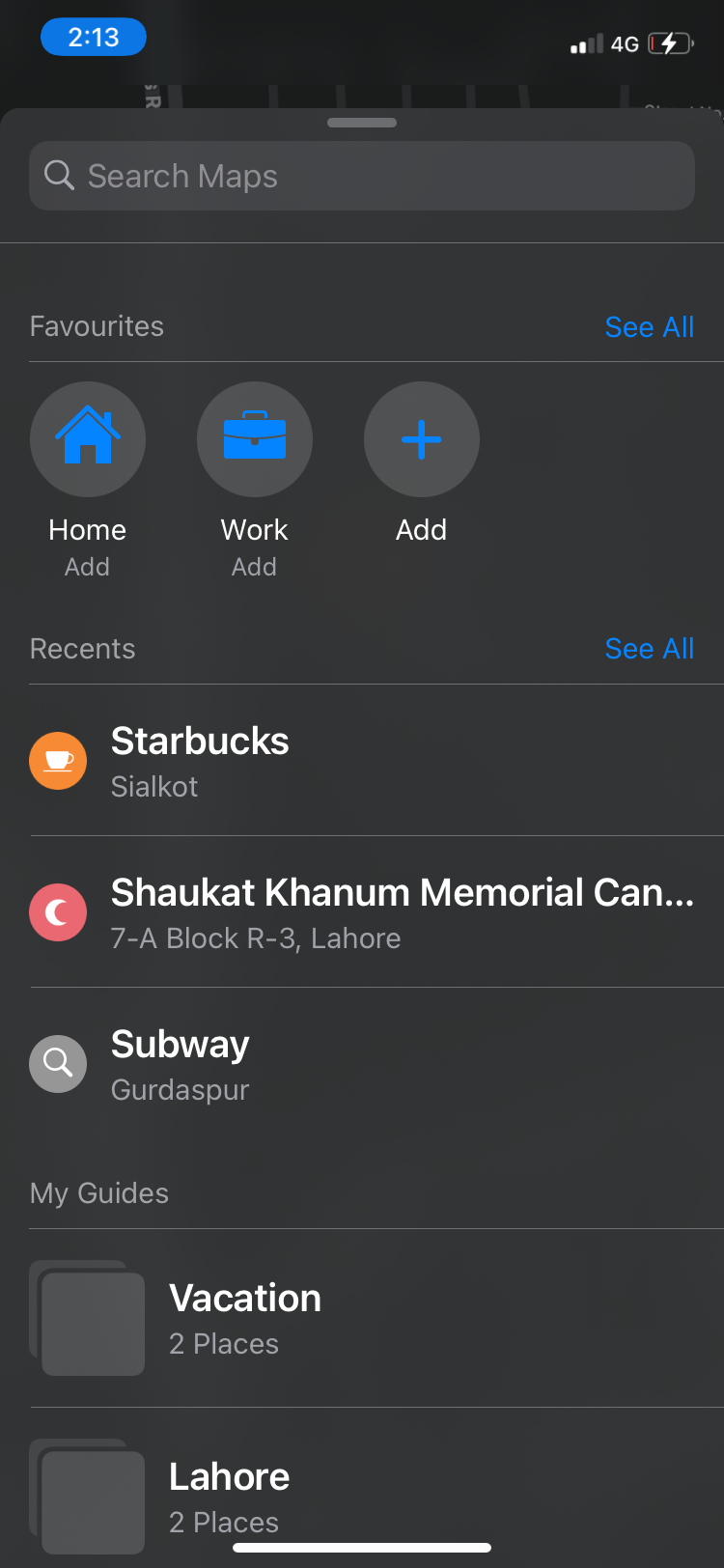The image depicts a smartphone screen with several elements visible. At the very top, a black banner shows a clock time of 2:13 in a small, blue oval. The phone is connected to a 4G network, with the signal strength indicator visible. The battery level is critically low, indicated by a red battery icon suggesting it's almost depleted.

Below the top banner, the screen is divided into distinct grey panels. The first panel features a search bar labeled "Search Maps." The second panel is titled "Favorites," with a "See All" option on the right, colored blue for easy visibility and interaction.

The third panel contains various icons, each accompanied by a label: a house icon symbolizing "Home," a suitcase icon representing "Work," and a plus icon indicating an add function. This panel also includes a clickable "See All" option, also highlighted in blue.

Following that is the "Recents" section, displaying recently searched locations: "Starbucks," marked by a coffee cup icon; a memorial place, denoted with a red moon icon; and a subway, indicated by a grey circle icon featuring a magnifying glass.

At the bottom of the screen is the "My Guides" section, showing two visible guides labeled "Vacation" and "Lahore."

Overall, the image provides a detailed look at the user's map and location interface, showcasing various functionalities and recent activities on their smartphone.